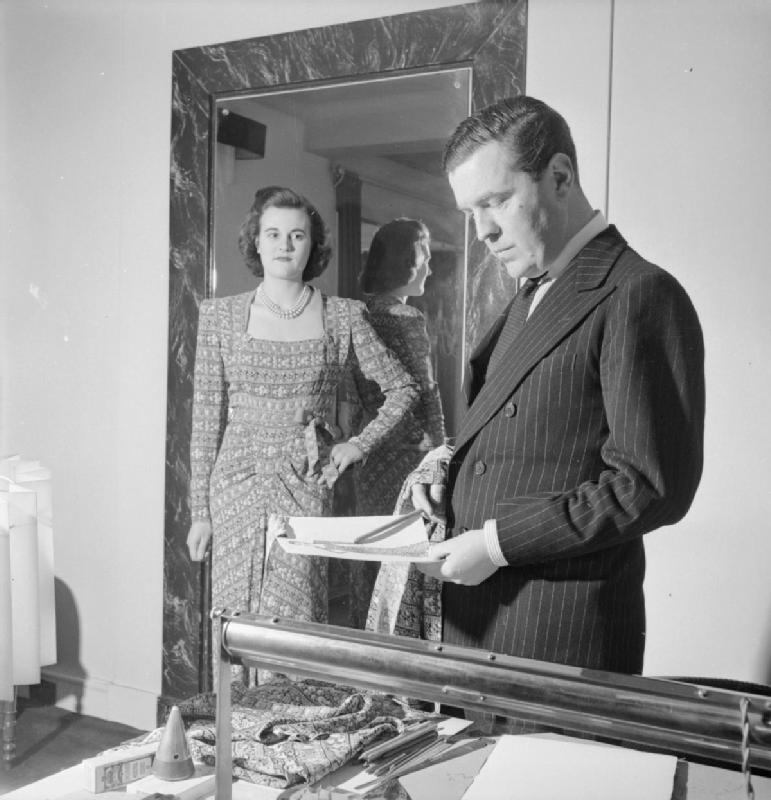This black-and-white photograph, likely from the 1940s, depicts an indoor scene centered around an older man and a younger woman. The man, positioned on the right, is intently studying a piece of paper while holding a pencil and a piece of textured fabric in his hands. He is dressed in a dark pinstriped business suit with a white shirt and black tie, his short hair slicked back. In front of him on the table are various items, including matching fabric and a cone-shaped tool. The woman, standing to the left, is dressed in a 1940s-style dress made of a similar material to the one the man holds. She wears a pearl necklace and has a period hairstyle. Although she stands in front of a framed marble mirror, she faces away from it, her indifferent expression directed toward the man. The background features white walls with visible scratches and dust marks on the film, indicating the photograph’s age.